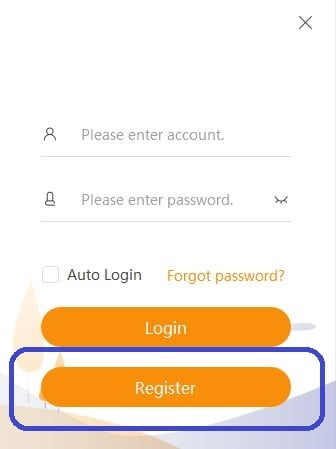The image appears to be a minimalist login screen, likely displayed on a mobile phone given its proportions. The top of the screen features a white background devoid of any traditional phone icons, with a simple 'X' placed in the upper right-hand corner. Below this, a line prompts the user to "Please enter account," paired with a subtle grey icon of a person on the left. Underneath, another line instructs "Please enter password," accompanied by a similar grey icon. Adjacent to this instruction, on the right, is a semi-circle with three radiating lines. Beneath the password line, the option to enable "Auto Login" appears in darker letters with a check box beside it. Next to this is "Forgot Password" highlighted in gold with a question mark.

Further down, the screen features a prominent orange "Login" button with gold text. Below this, another horizontally aligned orange button, outlined in blue, displays "Register." The background is adorned with a soft, watercolor-esque illustration of hills and trees in shades of orange and blue, adding a touch of artistic elegance to the otherwise simple interface.